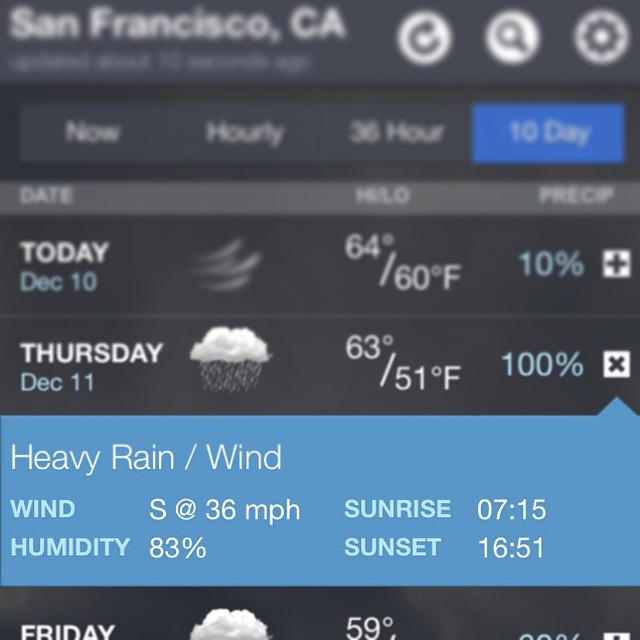The image depicts a weather forecast page for San Francisco, California, likely from a smartphone app or a web page. The top portion is somewhat blurred but shows the location "San Francisco, CA" with a black background. To the right, there are circular icons for reload, search, and settings. Below this, navigation tabs read "Now," "Hourly," "36 Hour," and "10 Day," with "10 Day" highlighted in blue, indicating it is selected. 

The forecast details presented include:

- **Today, December 10th:** Displayed with a wind icon, temperatures of 64°F (high) and 60°F (low), and 10% chance of precipitation.
- **Thursday, December 11th:** Displayed with a cloud and rain icon, temperatures of 63°F (high) and 51°F (low), and 100% chance of precipitation. An expanded section indicates heavy rain and wind, with wind speeds of 36 MPH, 83% humidity, sunrise at 7:15 AM, and sunset at 4:51 PM.
- Part of **Friday's** forecast is visible with a cloud icon and a high temperature of 59°F.

The overall interface includes column headers for date, high/low temperatures, and precipitation percentages, all displayed on a dark background with white text.